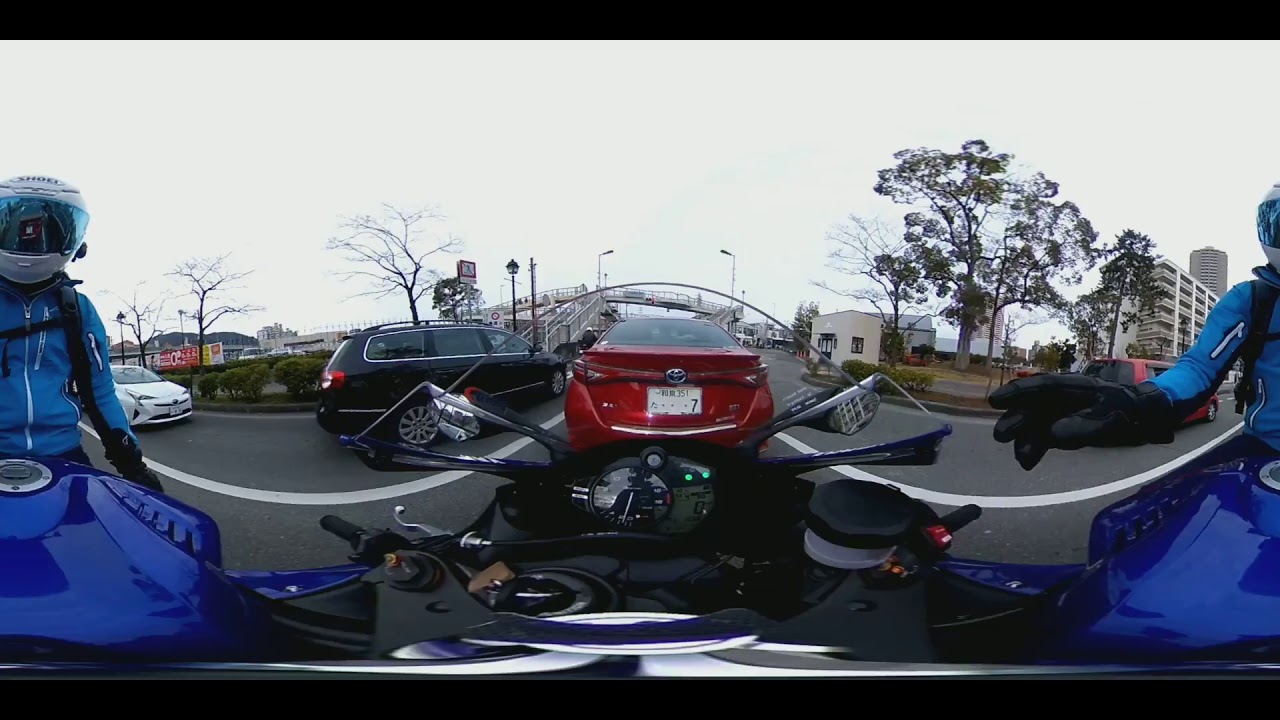In this dynamic 360-degree panoramic image, a motorcyclist wearing neon blue riding gear and a white helmet with a blue visor captures a photo from their blue motorcycle. The scene unfolds in a stretched-out format, displaying the same rider on both the right and left edges. The motorcycle has black handles and a shiny metallic blue body. The image reveals a of the scene from behind the handlebars and windscreen of the motorcycle. 

In front of the rider, several vehicles are visible: a distinctive red sedan with a foreign city license plate, a black SUV, and a white two-door car on the left. The road, marked with white stripes, stretches ahead under a hazy, cloudy sky. The background features trees, multi-story buildings, a distant bridge, and a highway overpass. The rider's right arm, clad in a big black glove, extends forward, possibly pointing or holding a GoPro camera. The level of detail suggests a busy urban setting, though the exact city remains unidentifiable.